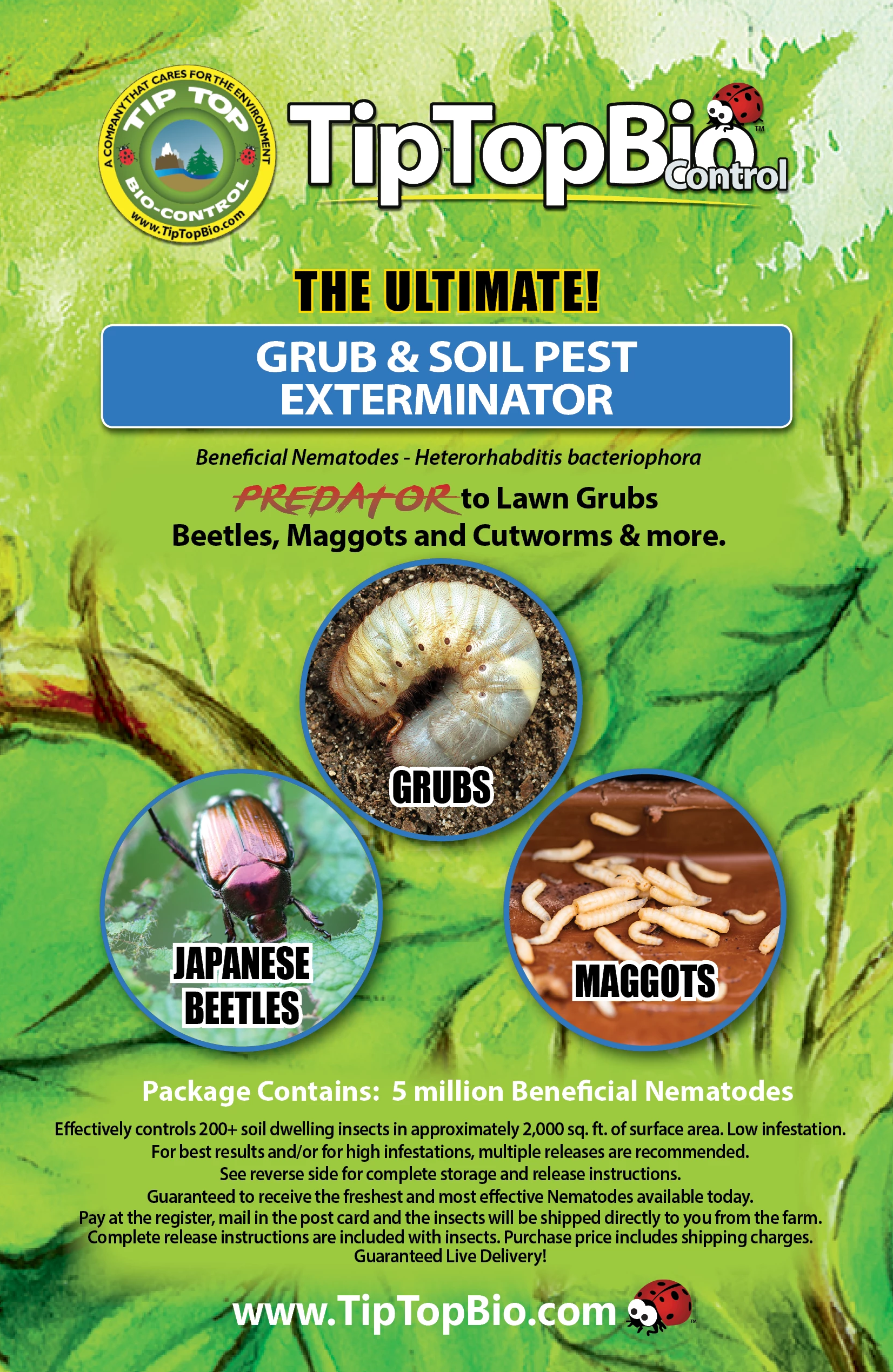This full-color, vertically rectangular advertisement image for a lawn care product titled "Tip Top Biocontrol" features vivid green tones with a backdrop of trees and shrubbery. The topmost section prominently displays the title "Tip Top Biocontrol" in white text against a black border, followed by the tagline "The Ultimate Grub and Soil Pest Exterminator" rendered in black text with a yellow border, and "Grub and Soil Pest Exterminator" in white text within a blue box. 

Beneath this title, the text reads "Beneficial Nematodes, Heterohabitatus Bacteriophora, Predator to Lawn Grubs, Beetles, Maggots, and Cutworms." This is supplemented by three circular photographs showcasing the pests: a shiny, metallic brown Japanese beetle labeled "Japanese Beetle," a whitish grub labeled "Grubs," and what appears to be a larvae labeled "Maggots." Further down, the image indicates that the package contains five million beneficial nematodes. At the bottom of the advertisement, there is a website URL, "www.tiptopbio.com," accompanied by a small ladybug image.